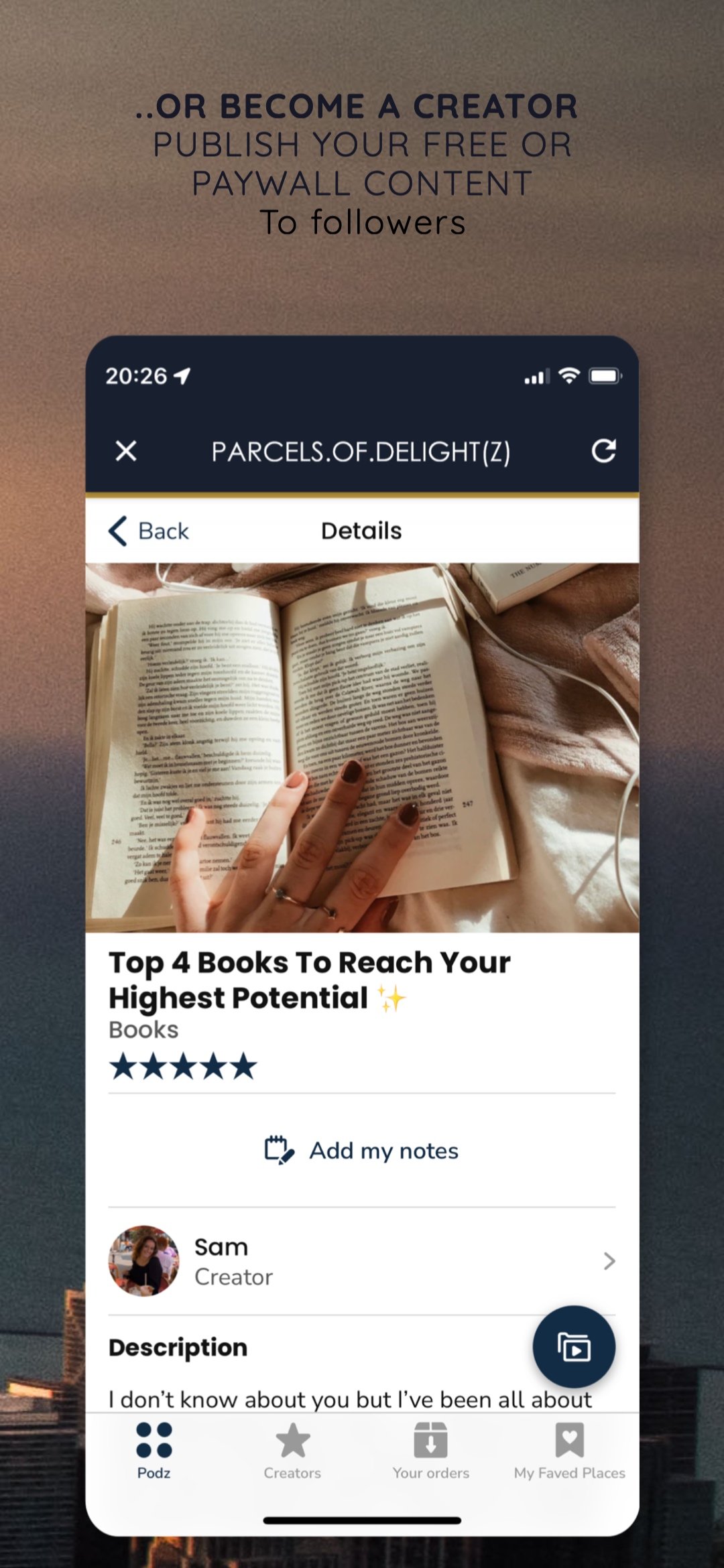A detailed caption for the described image could be:

"Screenshot of a user interface with a sky-themed background, featuring various interactive elements. At the top, bold text reads 'Become a Creator' alongside options such as 'Publisher', 'Free or Paywall Content to Followers'. The screen displays the time as '20:26'. An 'X' button labeled 'Parcels of Dr. Light' with a number '(2)' in parentheses appears, alongside refresh and exit buttons situated on the right and left respectively. Below, navigation buttons labeled 'Back' and 'Details' are present. The central section showcases an image of a woman reading a book, visible with her left hand on the book. There is a header stating 'Top 4 Books to Reach Your Highest Potential', followed by a five-star rating. Additional elements include an 'Add My Notes' button, the name 'Sam' labeled as the creator, and a brief description starting with 'I don't know about you, but I've been all about...'. At the bottom of the screen, four navigation dots are accompanied by tabs labeled 'Pods', 'Creators', 'Your Orders', and 'My Fave Places'."